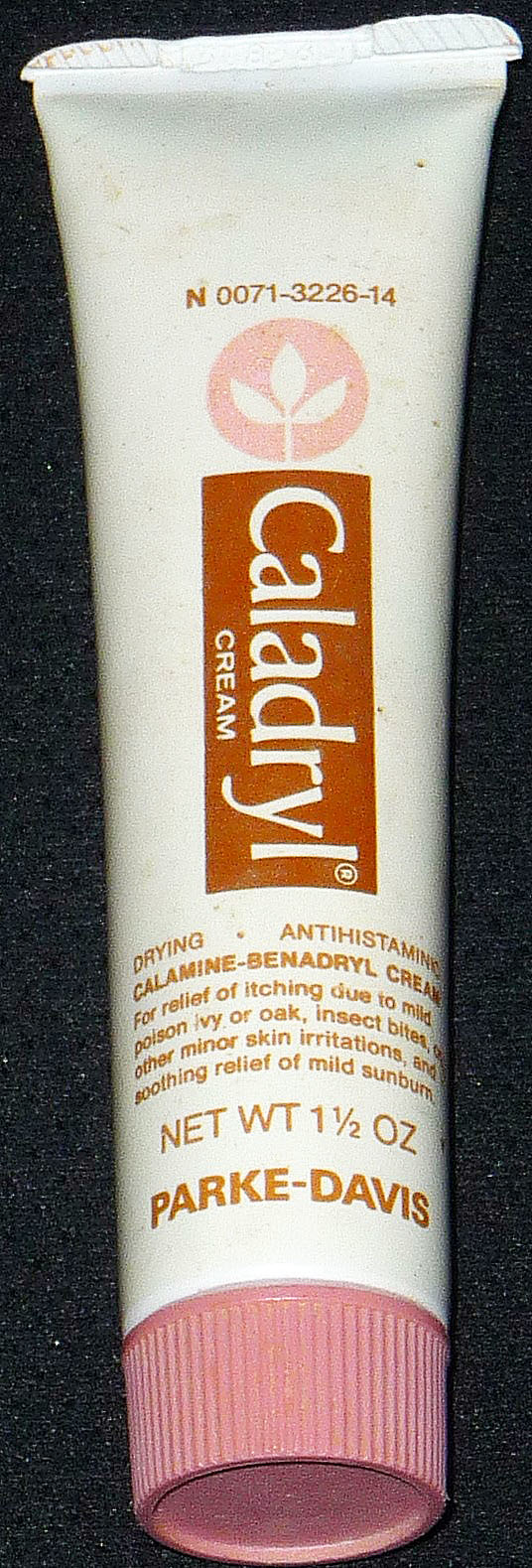The image depicts a white tube of Caladryl cream with a pink cap. The front of the tube prominently displays the name "Caladryl" in white letters on a vertical brown rectangle. Above this, there is a sequence of numbers: N0071-3226-14. Near the top of the tube is a logo consisting of a pink circle enclosing three white leaves. The bottom section of the tube provides a detailed description, indicating that the cream is a drying antihistamine calamine and Benadryl formula intended for the relief of itching due to mild poison ivy or oak, insect bites, other minor skin irritations, and mild sunburn. The net weight is specified as one and a half ounces. The manufacturer, Parke-Davis, is noted at the very bottom of the tube.